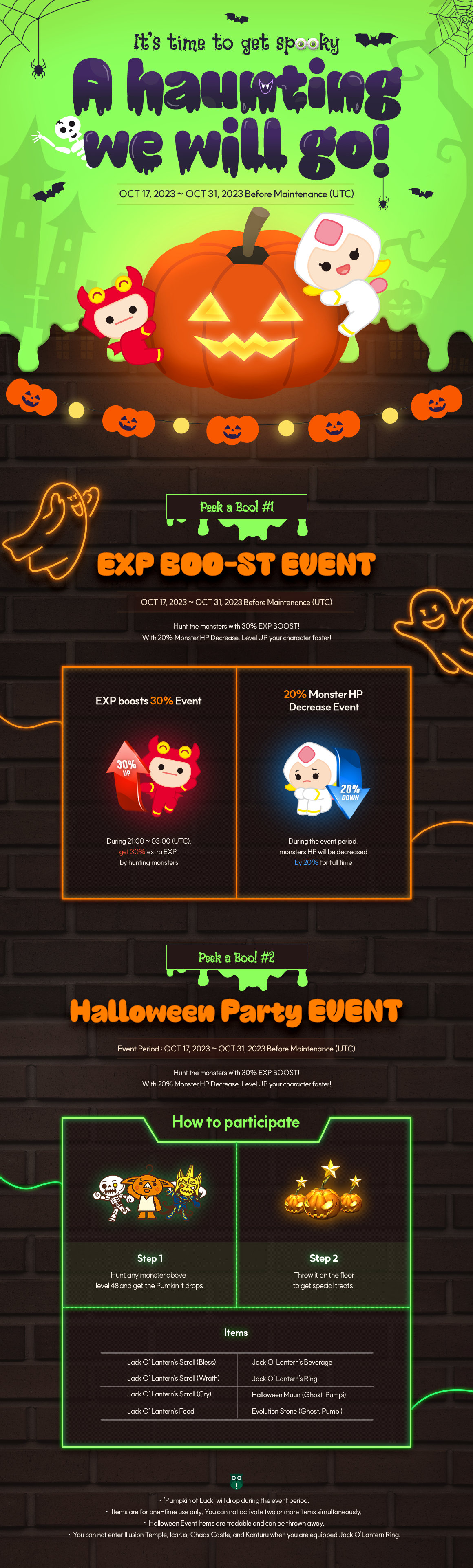A detailed and descriptive caption for the provided image would be:

"In this festive Halloween-themed image, a spooky scene is depicted against the backdrop of a grayish-black, brick building. The scene is centered around a carved pumpkin that glows with an eerie light from within, its face menacingly illuminated. Above it, text in orange announces an 'EXP Boost Street Event,' while adjacent text promotes a 'Halloween Party Event' with details on how to participate. The image is split into two main sections: the first showcases cartoon characters dressed in costumes, happily trick-or-treating; the second features three intricately carved pumpkins glowing with internal lights, each topped with decorative stars. The entire composition captures the essence of Halloween, blending the excitement of trick-or-treating with the haunting beauty of jack-o'-lanterns."